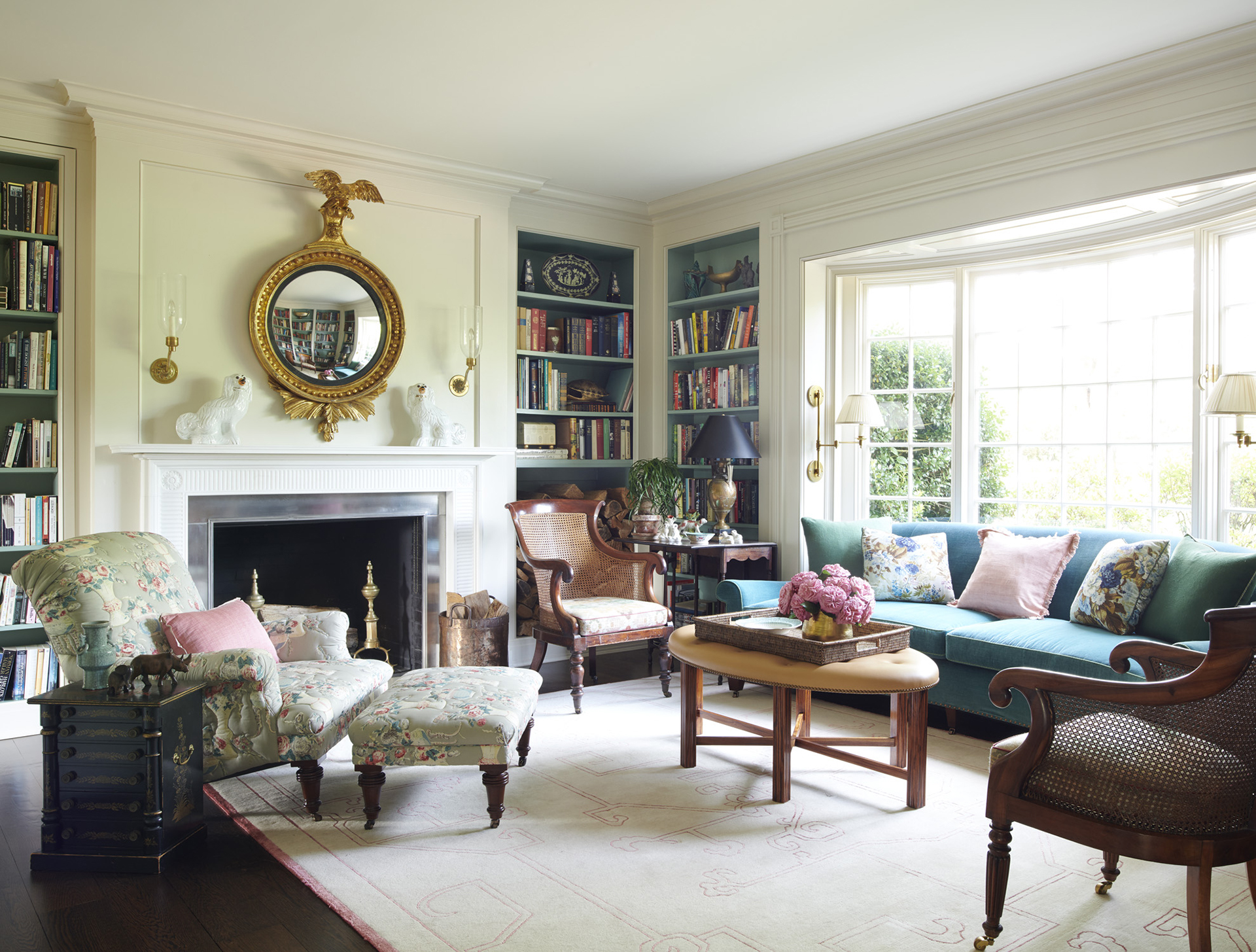The photograph captures an elegantly furnished living room exuding sophistication. Dominating the right side, a large bay window adorned with white trim and divided panes floods the room with light. Flanking the window are two lamps with white shades. In front of the window is a bluish-green couch embellished with three pillows. A unique coffee table, featuring a cushion top and dark wood legs, serves as a central piece, along with a tray holding a vase of pink flowers.

Adjacent to the couch, on either side, are two wicker chairs with brown to cherry-colored wood and white seats, adding a touch of rustic charm. To the left, against the opposite wall, stands a white fireplace with intricate grayish-pink tile work, crowned by a resplendent gold mirror with an American Eagle motif. Perched on the mantel are two porcelain dogs, white with gold detailing, adding a whimsical touch. 

The room boasts three built-in bookcases filled with an extensive collection of books, emphasizing the intellectual character of the space. A floral green upholstered armchair with a matching footstool, adorned with a pink pillow, invites relaxation. Complementing the classical decor, a lamp with a gold base and purple shade rests on a table beside one of the bookcases. The floor is dressed in a plush white rug with pinkish-colored trim and design, tying together the room's luxurious and refined aesthetic.